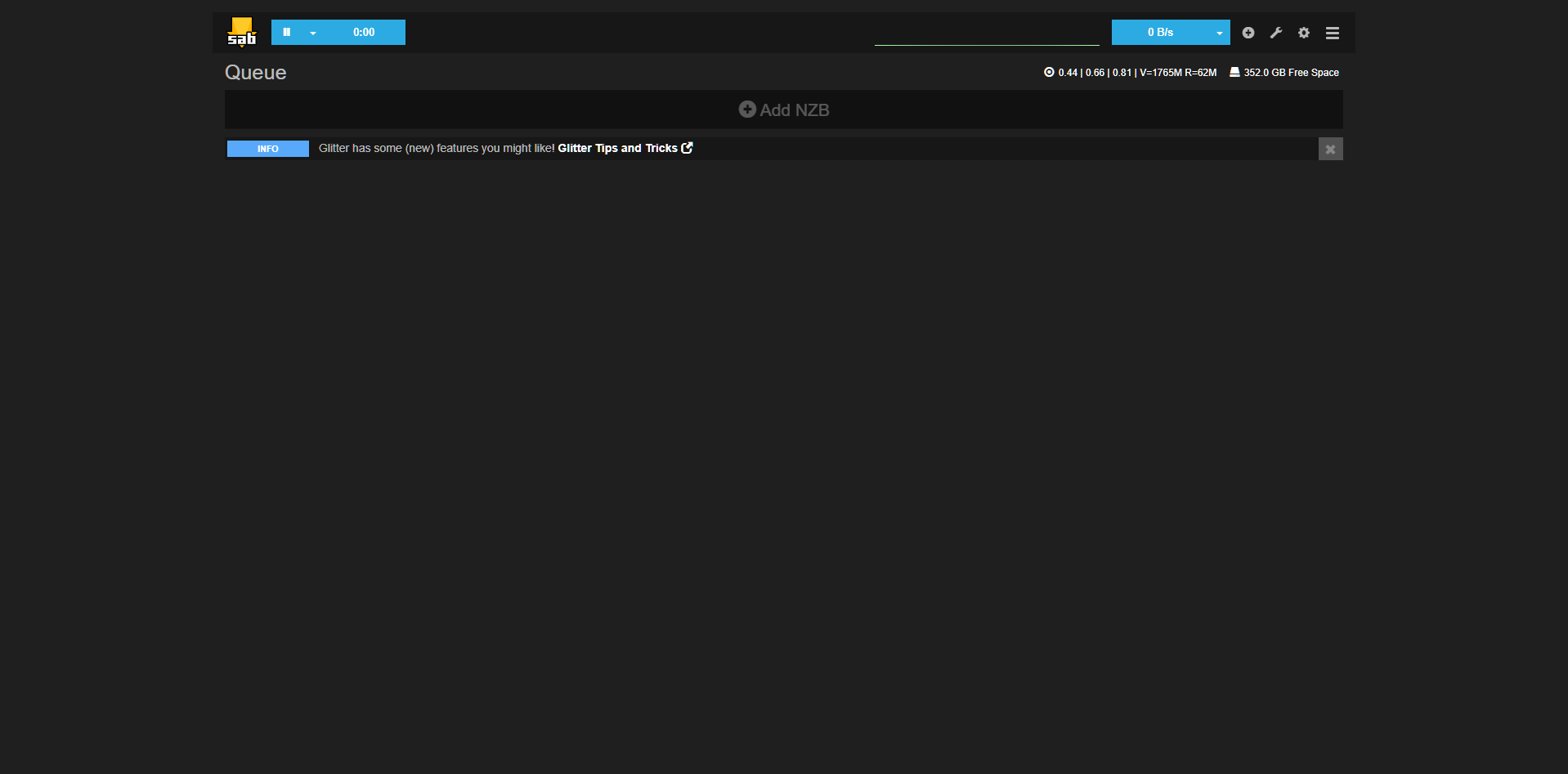This is a screenshot of a website or application displayed on a computer screen with a dark gray background. 

- At the top left corner, there is an orange arrow pointing downward with the letters "SAB" superimposed on it.
- Adjacent to this logo, there is a bright blue button featuring white icons that include a pause symbol on the left, a downward arrow in the middle, and the time display "0:00" on the right. 
- To the right of this button is an area of negative space, followed by a thin green search bar that is underlined in light green.
- Right next to the search bar is another bright blue button labeled "0B/S" with an accompanying downward arrow in white text.
- Further to the right, situated on the gray header section, is a series of white icons including a circle with a gray plus sign, a wrench, a cog, and three vertically-stacked lines.

Beneath the SAB logo, there's the letter "Q" in white text.

- On the far right side of the page, there is a section displaying a white target symbol followed by the numbers 0.44, a vertical line, 0.66, another vertical line, 0.81, another vertical line, and the text "V=1765M, R=62M". 
- Just below this, a hard drive icon is displayed alongside the text "352.0GB free space".

Further down the page:

- A horizontal black bar spans almost the entire width of the screen and contains a gray circle with a dark gray plus sign. This bar also features the text "Add NZB".
- Below this bar, toward the left side, there is a blue button labeled "Info" in white text.
- To the right, a notice reads "Glitter has some new features you might like" in white text on a dark gray background, followed by the words "Glitter Tips and Tricks" and an external link icon.
- To the right of this notice, there is a light gray square with a lighter gray "X" in it.

This detailed, organized description captures all the key visual elements and their respective positions within the screenshot.